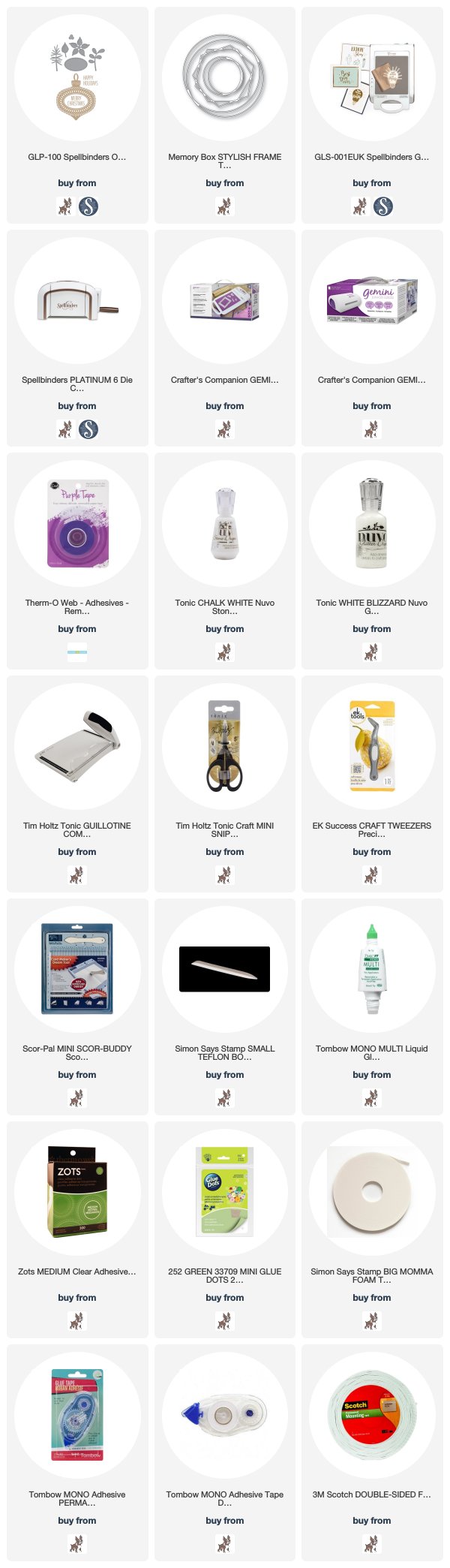Here is a cleaned-up and detailed caption for the image:

The website image showcases a neatly organized grid of 21 products available for purchase, arranged in three columns of seven. Each product is individually displayed within a portrait-oriented rectangle featuring a light gray background, separated by thin white lines. 

At the top of each rectangle, there is a distinct white oval housing the product image. Directly below the image, the product name is written in tiny, somewhat hard-to-read text, followed by the bold text "Buy from." Below this, various logos indicate the sellers, including a recurring small dog logo and a blue circle with a white "S."

Notable products include:

- **Upper Left Corner:** A collection of possible Christmas ornament stickers featuring designs such as a gold-colored ornament, a gray star, a gray oval, and gray leaves.
- **Middle Column, Fourth Row:** A pair of black-handled scissors with short tips, showcased within a store-style hanging box.
- **Lower Right Corner, Second from Bottom:** A rolled circle of white material resembling old whiteout tape or sticky tape, tightly wrapped in a white circle.
- **Bottom of First Column, Second from Bottom:** A black and green box labeled "ZOTZ."
- **Bottom Center of the Middle Column:** A product that appears to be Krazy Glue, housed in an identifiable packaging.
- **Middle Column, Third from Top:** A bottle possibly containing whiteout.
- **First Column, Fourth from Top:** An open paper cutter with the word "guillotine" beneath it, indicating its function as a paper trimmer.

These items, along with others in the grid, represent various non-paper supplies typically found in a paper supply store.